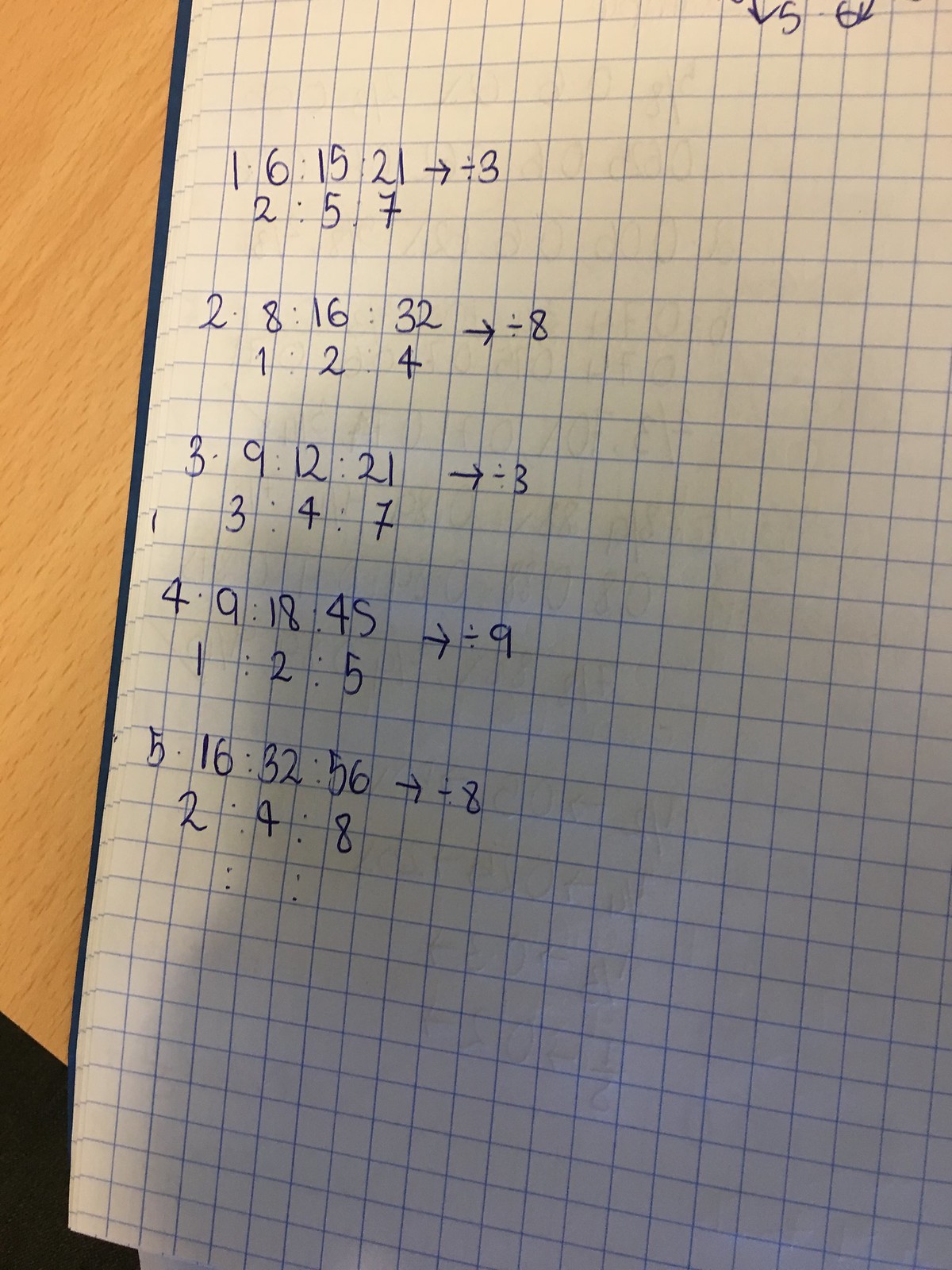This photograph showcases the left-hand side of a graph paper notebook, presumably used for math homework. The notebook, with its black cover slightly visible around the edges, features a series of numerical problems written in blue ballpoint pen. The page displays problems numbered from 1 to 5, with the first one illustrating a sequence: "6:15:21" followed by an arrow pointing to a division symbol and "3." Directly beneath these numbers, there is a line reading "2:5:7." In the background, on the left side of the image, a medium bright wood-colored tabletop is discernible, adding contrast. A black object, possibly an arm or an indistinguishable part of the background, appears in the bottom left corner. The detailed segmentation of the grid paper and the clear, neat handwriting suggest an organized approach to problem-solving.